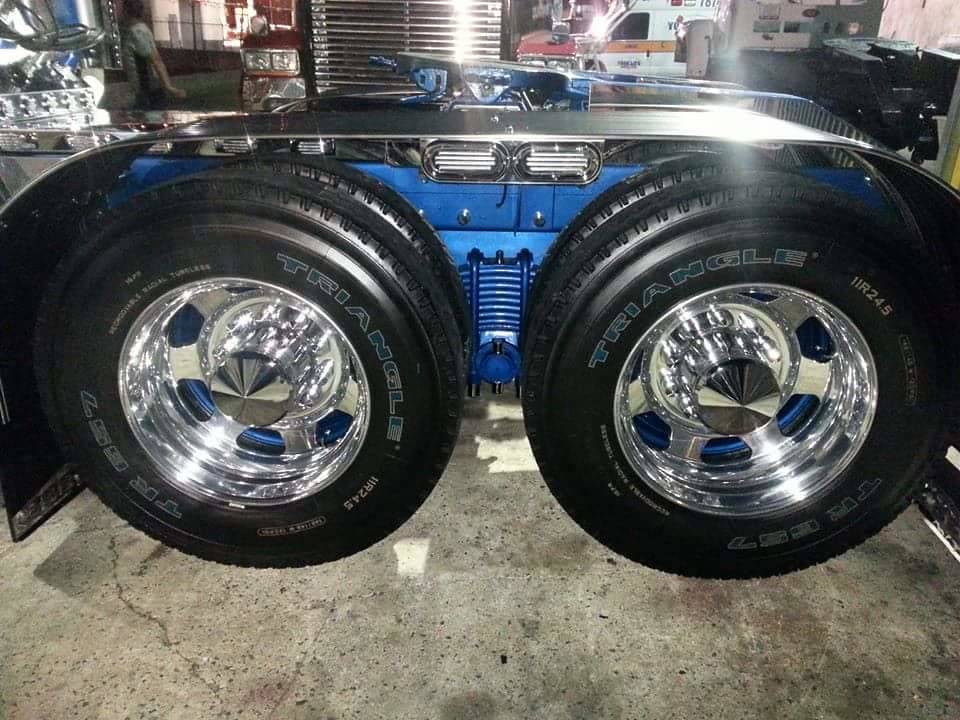This image captures a detailed view of two enormous truck tires prominently labeled with "TRIANGLE" in white font with blue accents. The tires, marked with product identifiers "IIR245" and "TR357," have gleaming silver hubcaps at their centers. They are mounted on a blue metallic rectangular structure, likely part of a truck that is mostly out of the frame. A curved silver cover stretches over the top, shielding the front and rear of these tires.

The scene is set in a machine shop or a garage, evident from the dirty white and gray speckled concrete floor and the presence of tool shelves and various machinery in the background. An ambulance and the front of another truck are also discernible in the distance. A person is visible in the upper left corner, though blurry due to the distance. The overall clutter and environment suggest an active work area focused on vehicle maintenance or repair.